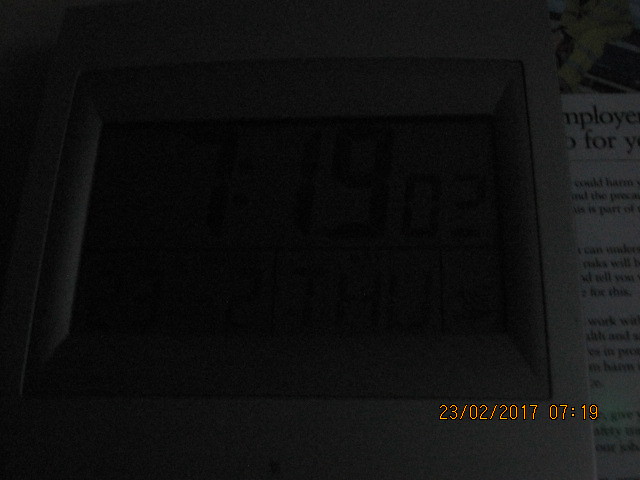This photograph captures a dimly lit computer screen, shrouded in darkness. The screen's display features a sequence of concentric rectangles: a central black rectangle framed by a gray one, and an outer, lighter gray rectangle, all enveloped in shadow. In the lower right-hand corner of the screen, digital text reads "23-02-2017-07-19." Behind the computer monitor, there is a visible clipping, possibly from a magazine, poster, or newspaper. This clipping includes fragmented text with the discernible phrases "could harm," part of the word "employee," and "for."